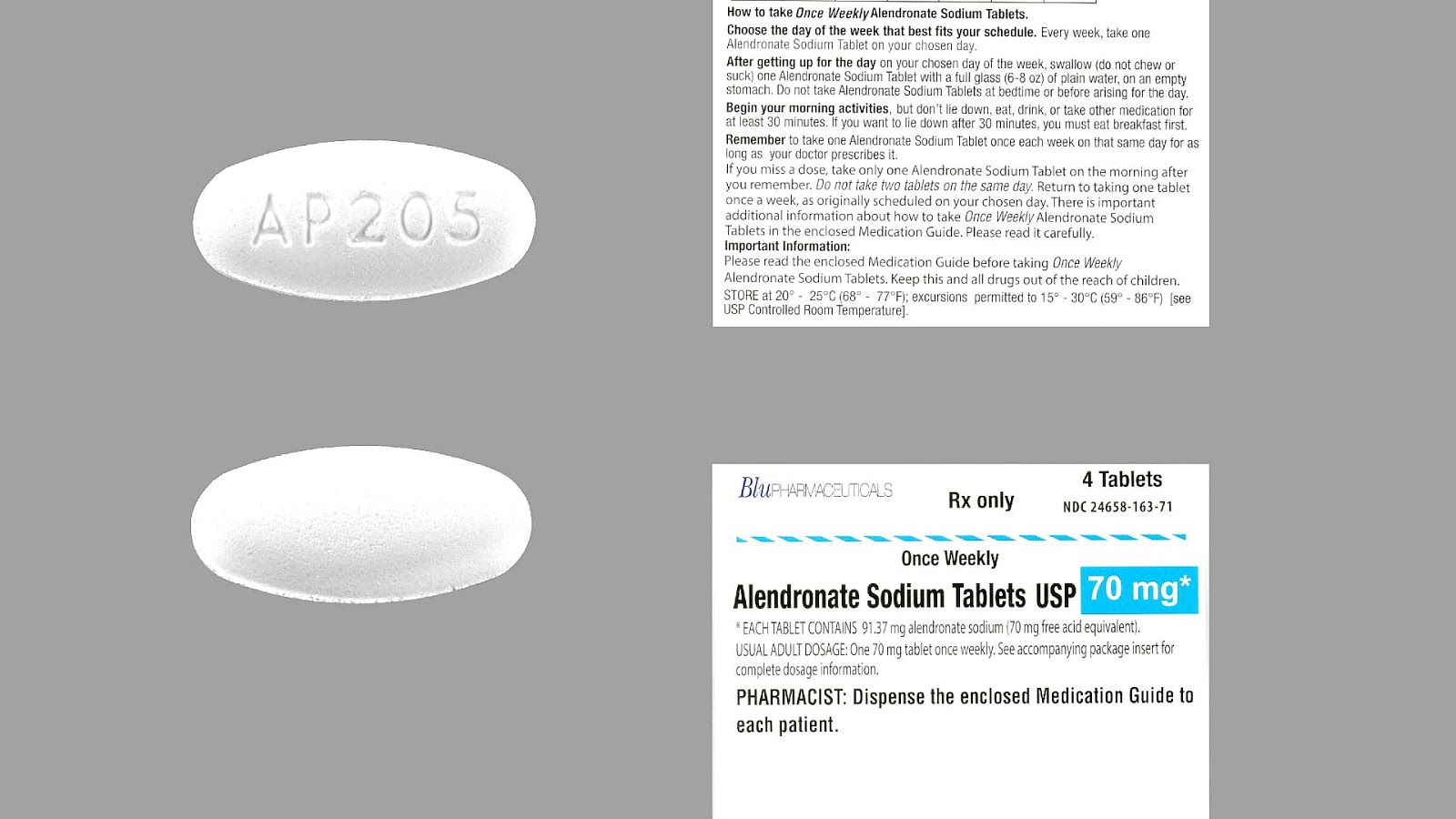The image features a grey background with a pill on the left side. The pill is oblong and white, with "AP-205" inscribed on its top half, while the bottom half remains blank. To the right of the pill, a detailed text box provides instructions on how to take a once-weekly Alendronate Sodium tablet. The instructions advise choosing a day that best fits the user's schedule and consistently taking one tablet on that chosen day every week.

Upon waking on the chosen day, the user should swallow the tablet whole with a full glass (6-8 ounces) of plain water on an empty stomach. The instructions emphasize not chewing or sucking on the tablet. Taking the tablet at bedtime or before arising is discouraged. After taking the tablet, the user should begin their morning activities and avoid lying down, eating, drinking, or taking other medications for at least 30 minutes. Breakfast should be consumed before lying down if needed after this initial 30-minute period. A reminder at the end of the text prompts the user to continue this regimen for as long as prescribed by their doctor.